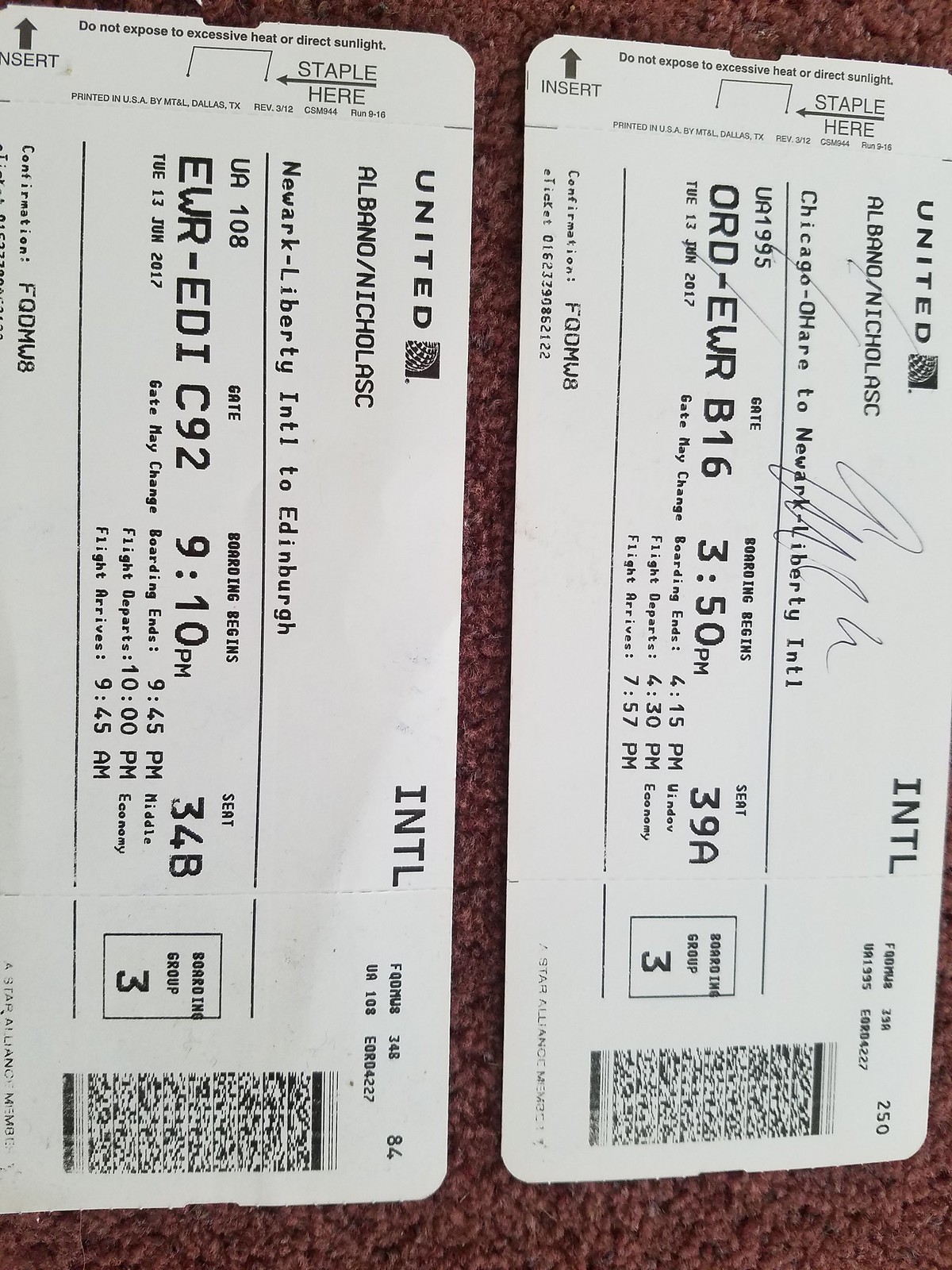The image is a tall, vertical photograph featuring two airplane tickets laid side by side on a brown, fluffy rug. Both tickets are rectangular with curved corners and positioned centrally in the image. The tickets are for the same traveler, Albano Nicholas C. The ticket on the right lists a flight from Chicago O'Hare to Newark Liberty International, with flight details ORD-EWR-B16, departure at 3:50 p.m., seat 39A, and boarding group 3. The ticket on the left details the next leg of the journey, from Newark Liberty International to Edinburgh, identified by the flight code EWR-EDI-C92, boarding at 9:10 p.m., seat 34B, and also in boarding group 3. Each ticket features several rows of numbers, times, dates, and rectangular barcodes at the bottom. The setting appears to be indoors, and the tickets fully occupy the image against the soft, textured backdrop of the carpet, suggesting they are casually scattered on the floor, poised for a snapshot by the traveler preparing for their trip to Scotland.